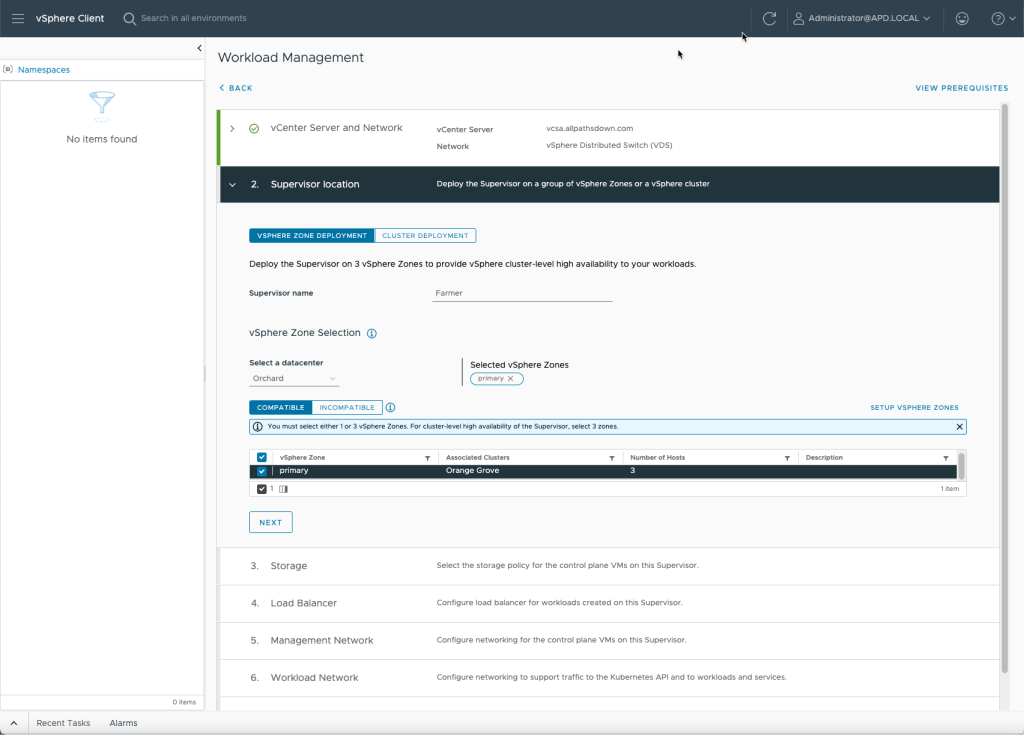This detailed description accompanies a screenshot of a vSphere Client web page interface. The web page features a clean, white background topped with a dark grey banner. In the upper left corner of the banner, the text "vSphere Client" stands out in white against the grey. Adjacent to this text, a search bar is prominently positioned, while the upper right corner of the banner hosts a reload button and a dropdown menu.

The primary section of the image showcases a heading that reads "Workload Management." Directly beneath this heading is a white box accentuated by a vertical green line, labeled "vCenter Server & Network." Following this, a thin grey box identifies the section as "Supervisor Location."

The first detailed section is titled "vSphere Zone Deployment Cluster Deployment." It includes a brief explanation: "Deploy the supervisor on three vSphere zones to provide vSphere cluster level high availability to your workloads." Below this description, input fields are available for "Supervisor Name" and "vSphere Zone Selection."

The lower portion of the main section is divided into four labeled columns, specifically "Storage," "Load Balancer," "Management Network," and "Workload Network," corresponding to numbers 3, 4, 5, and 6, respectively. 

Additionally, the left side of the image features a vertical column containing an icon resembling a funnel, along with the text "No Items Found." The bottom left corner of the interface displays the taskbar with sections labeled "Recent Tasks" and "Alarms."